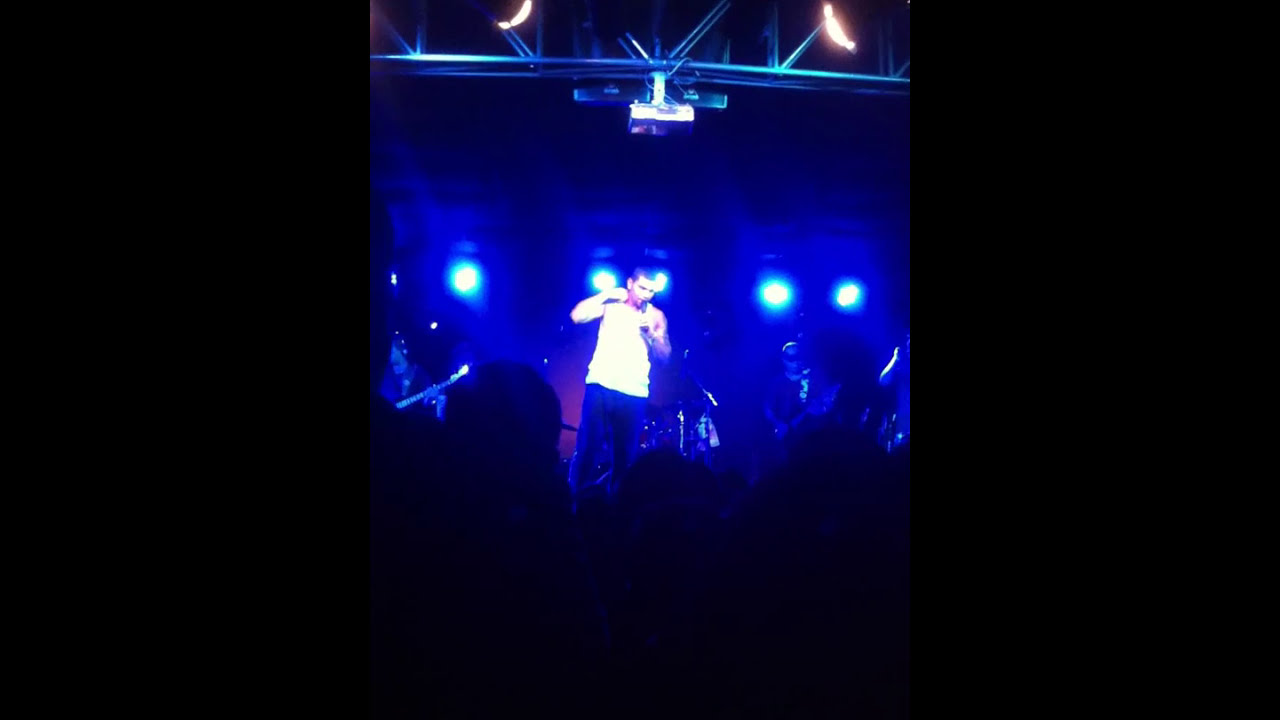The image captures a dynamic moment on stage with a young man front and center, holding a microphone in his left hand while his right hand is near his neck. His short dark hair matches his casual outfit of a white t-shirt and dark-colored pants. Behind him, the band includes musicians with guitars to both his left and right, and a drum set further in the background. The stage is illuminated by five orbs of light, creating a blue hue that bathes the scene in a cool tint. Framework and additional lights can also be seen at the top of the stage. The audience, partially visible in the foreground, watches intently, adding depth to the image, which appears dark overall except for the well-lit stage. The moment is captured with the feel of a live performance, possibly intended for social media sharing.